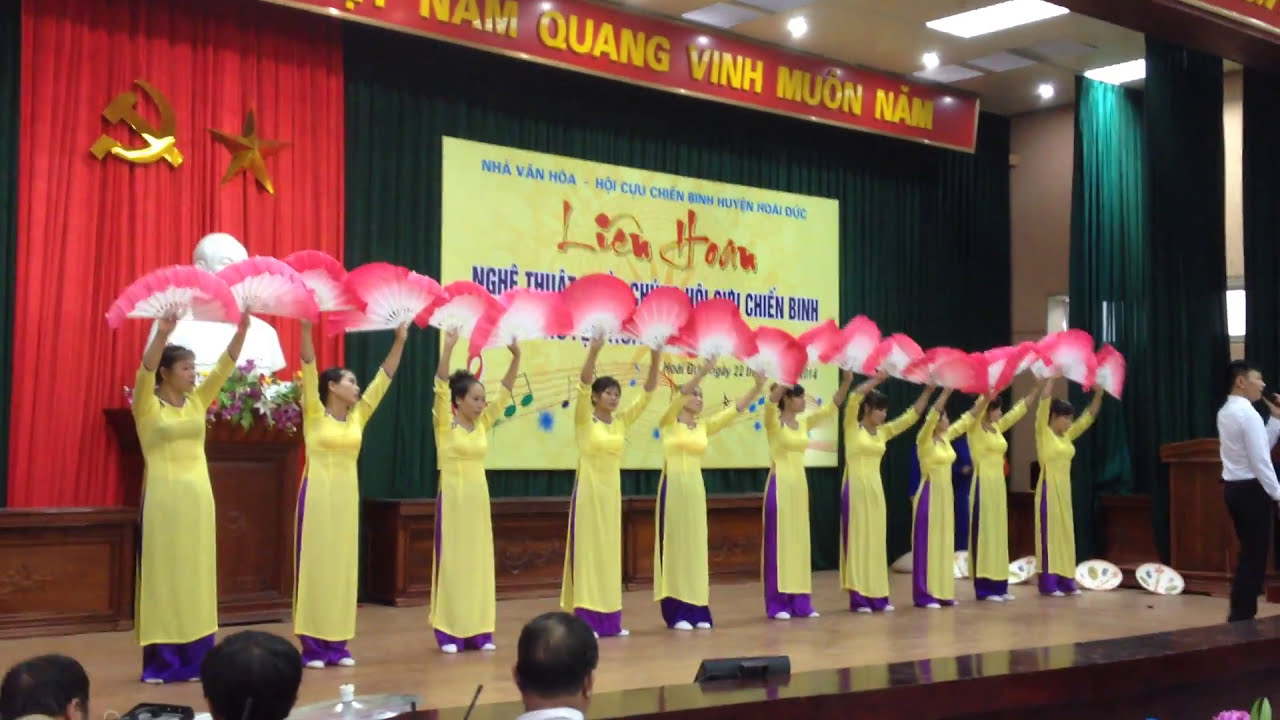The image depicts a group of approximately 10 very thin women on a small stage, all dressed uniformly in light yellow dresses paired with vibrant purple pants and white shoes. Each woman is positioned in a line at the front of the stage, arms raised uniformly above their heads, each holding a pink and white fan. In front of the stage stands a man in a white shirt and black pants, holding a microphone and speaking to the audience. Behind the group, a large yellow sign with Vietnamese lettering is prominently displayed. The backdrop includes dark curtains with a distinct red section adorned with the gold Communist star and hammer and sickle. Additionally, a bust accompanied by flowers on a podium is visible to the left. Above the stage, there is a red sign with more yellow Vietnamese text. The image also captures the backs of three audience members' heads at the bottom left of the frame, looking attentively at the stage.